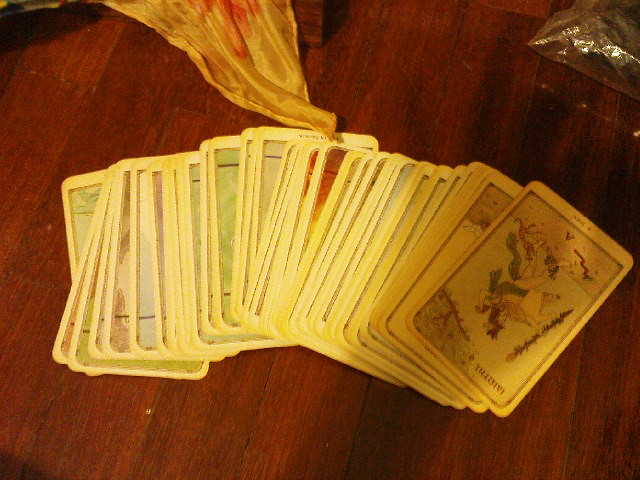An overhead photograph captures a collection of vintage-looking cards spread out on an aged, deep brown wooden table, marked by numerous scratches and imperfections. The cards, displaying muted white backgrounds, exhibit signs of weathering with yellowed or burnt-looking edges. Arranged from left to right, the cards draw the viewer's eye to the foremost card on the right. This card features a cartoonish depiction of a woman adorned with a shawl around her shoulders and a green one around her waist. She holds a stick and a staff, and a branch laden with fruit hovers above her head. Adding extra details to the scene, a plastic bag is seen just above the cards, and a yellow cloth lies in the upper left corner of the image, contributing to the rustic and eclectic atmosphere.